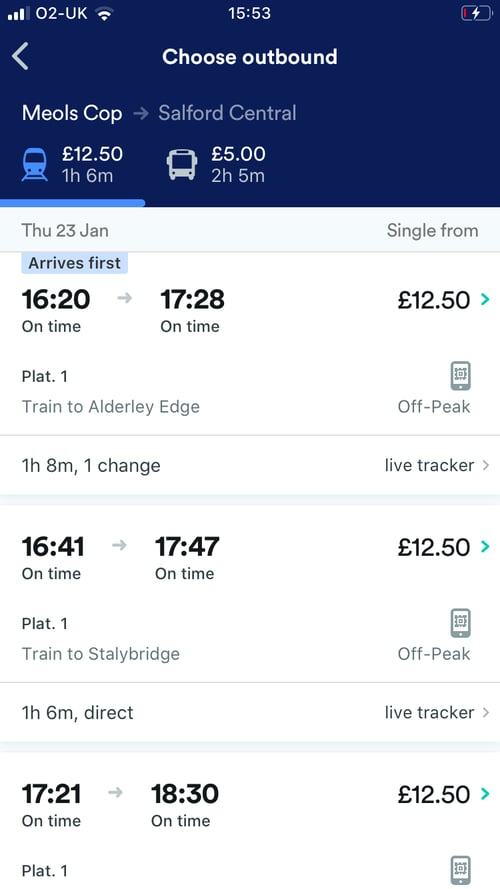The image is a screen capture from a cell phone application displaying various train ticket options. In the upper right corner, there is a battery charging symbol indicating a low battery percentage, highlighted in red. To the left, the center of the screen prominently displays the time, 15:53. On the far left corner, the phone shows three bars of cell coverage with "02-UK" next to it and two bars of Wi-Fi coverage.

The top banner is dark blue with white text that reads "Choose outbound" accompanied by a left-pointing arrow. Below, the route is specified as "Melos Cop" with a right-pointing arrow leading to "South Ford Central." An icon of a train appears below this route header, and next to it, the fare is listed as £12.50 with a journey duration of one hour and six minutes.

Underneath this header, the screen lists different train ticket options:

1. **First Option:**
   - **Date:** Thursday, 23rd January
   - **Ticket Type:** Single form; arrives first
   - **Departure:** 16:20 (on time)
   - **Arrival:** 17:28 (on time)
   - **Fare:** £12.50
   - **Platform:** 1 
   - **Route:** Train to Alderley Edge, off peak
   - **Duration:** One hour and eight minutes
   - **Transfer:** One change
   - **Feature:** Live tracker available

2. **Second Option:**
   - **Departure:** 16:41 (on time)
   - **Arrival:** 17:47 (on time)
   - **Fare:** £12.50
   - **Platform:** 1
   - **Route:** Train to Sally Bridge, off peak
   - **Duration:** One hour and six minutes
   - **Feature:** Direct journey with live tracker

3. **Third Option:**
   - **Departure:** 17:21
   - **Arrival:** 18:30
   - **Fare:** £12.50